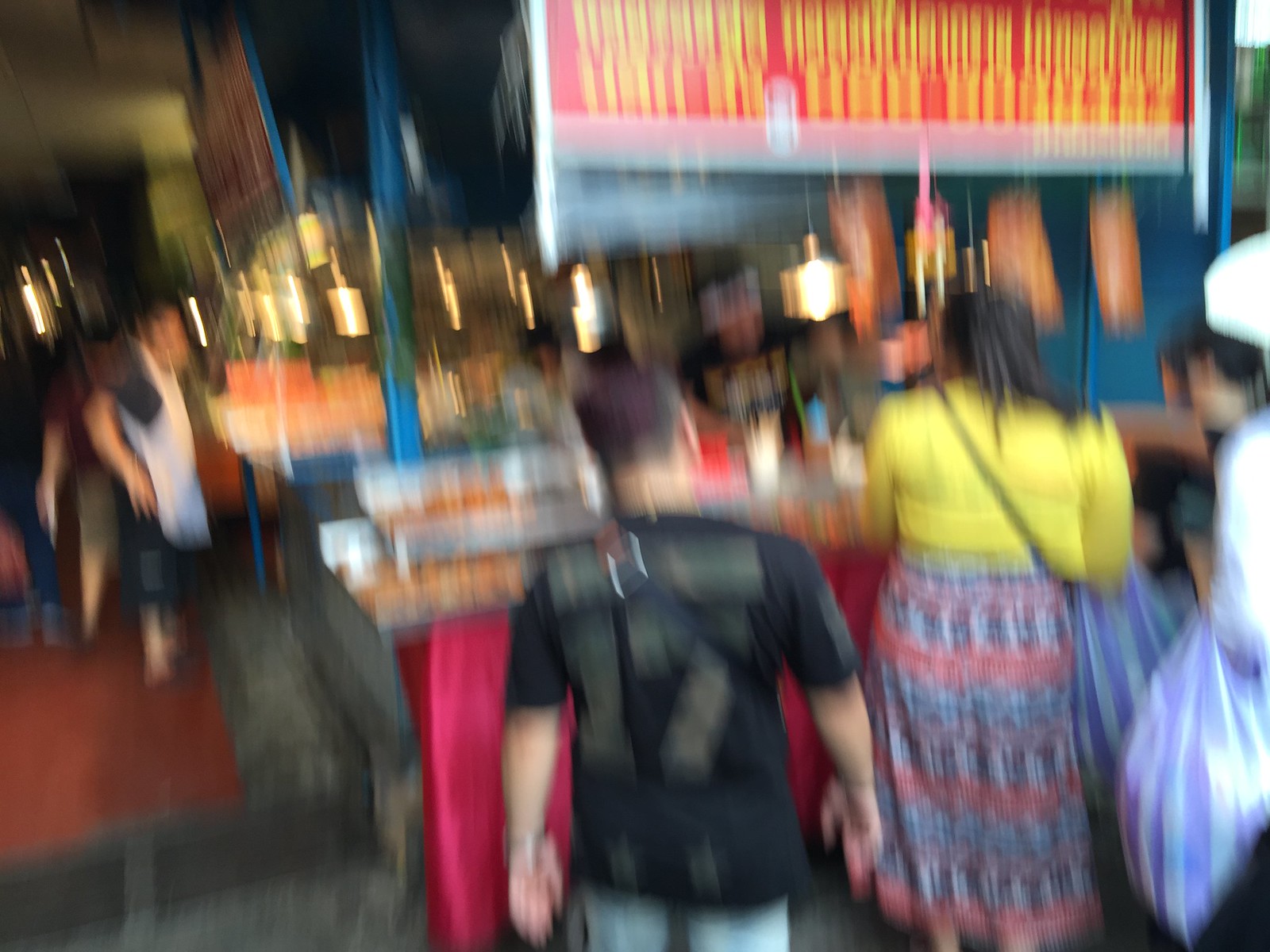In this extremely blurry nighttime photograph of what seems to be a bustling indoor market or festival, we can see around six or seven people amidst various booths. At the forefront, under dim, low-light conditions that resulted in a fuzzy, motion-affected image, stand three individuals with their backs to the camera. They appear to be at a food stall adorned with a red sign featuring yellow print.

The closest person on the left, identifiable by their yellow top and black strap, has dark hair tied in a ponytail, and they are wearing a distinctively patterned skirt colored in blue and red lines with a bluish-gray section. This person also carries a bag. Next to them is a shorter individual in jeans and a black shirt bearing the gold number 17 on the back along with indiscernible text. Further off to the left in the image, partially visible, stands another person in a white apron and blue shorts.

The table at the food stall is draped with a silky red sheet, and the area features a reddish-brown floor with gray patches in the foreground. The image conveys the lively, chaotic essence typical of a food market or festival, even though its blur obscures finer details.